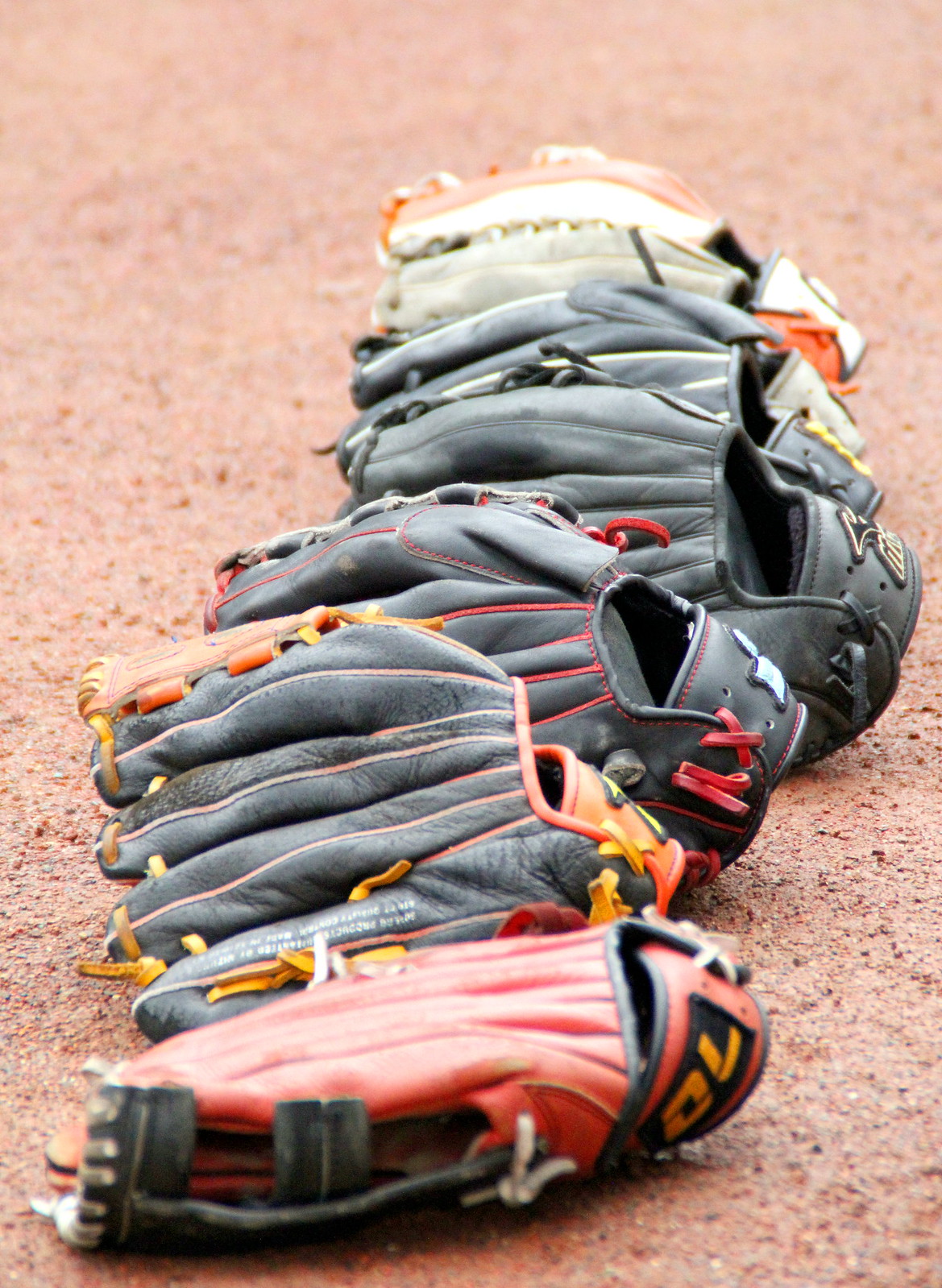This vibrant, vertically-oriented outdoor photograph captures a row of baseball gloves meticulously arranged on a reddish, textured surface typical of a baseball field. The gloves, which appear to be catcher's mitts made of worn, textured leather, exhibit various colors and stitching. The lineup starts at the bottom forefront with a bright brown glove displaying the number 70 in yellow font, followed by an old gray glove. Moving upward, three black gloves appear sequentially, then a black glove with red stitching, another black glove with brown stitching, and finally a brown glove at the very top. Each glove is positioned with its fingers pointing to the left and its wrist section to the right, creating a striking visual path that leads the viewer's eye from the front towards the background center. The photograph is bathed in bright sunlight, giving it a reddish or pink hue and casting detailed shadows that highlight the gloves' textures and intricately woven laces, making the scene both dynamic and nostalgic, reminiscent of a moment captured on a bustling baseball field.